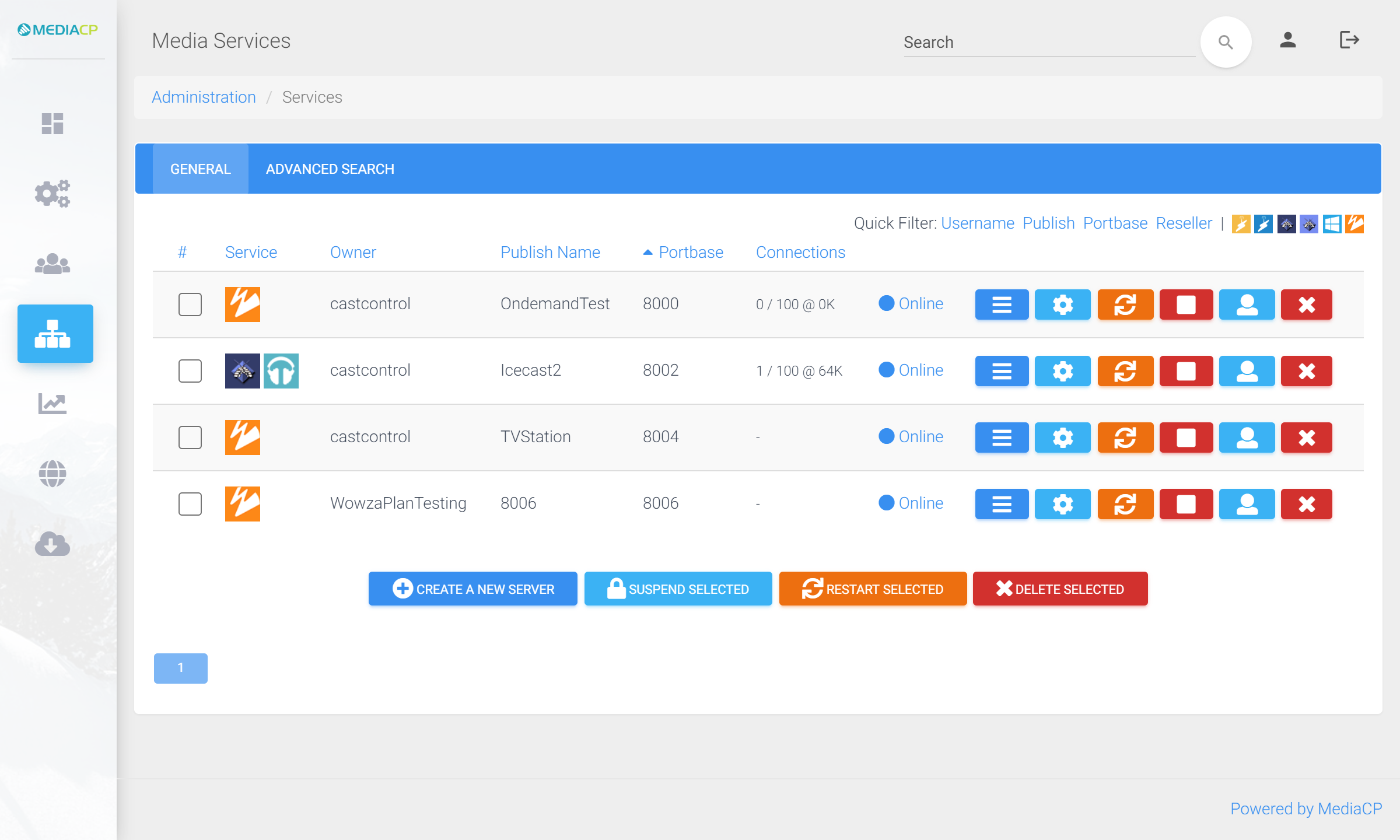The image depicts a light gray administration window labeled "Media Services." Below the main title, it reads "Administration/Services." A blue bar beneath this provides two tabs: "General" and "Advanced Search." Displayed in the window are four available services, each detailed with the following columns: Service, Owner, Publish Name, Port Base, and Connections. At the bottom of the window, there are several action buttons: a blue "Create a New Server" button, a light blue "Suspend Selected" button, an orange "Restart Selected" button, and a red "Delete Selected" button.